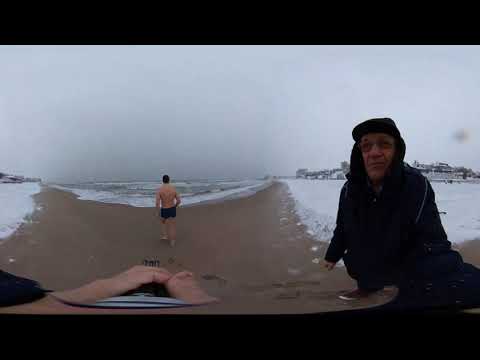This photograph captures a winter beach scene under a cloudy, overcast sky. The beach, covered in brown sand with patches of snow, stretches out toward a large body of water, possibly an ocean or a lake. Gentle waves roll in, frothy with white bubbles. In the middle distance, a man wearing only shorts walks resolutely toward the chilly water, seemingly unfazed by the cold. In the lower right corner of the image sits the person who took the photo, dressed warmly in a black cap and dark clothing that includes a thick hoodie for protection against the cold weather. To add depth to the scene, small buildings are visible in the background behind the photographer, and horizontal black strips frame the top and bottom of the image, enhancing the contrast of this cold, serene landscape.